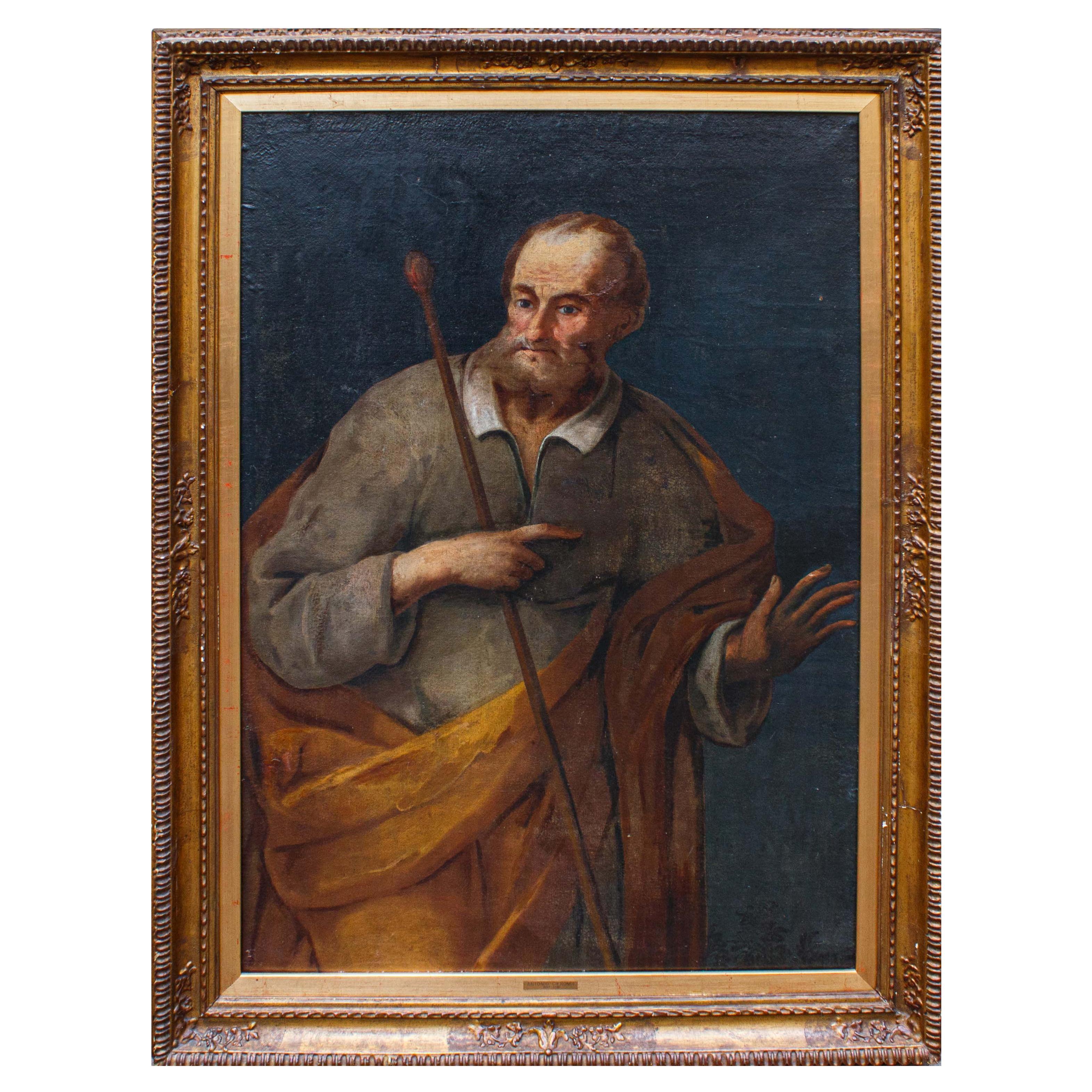This painting features a detailed portrait of a man encased in an ornate, light-colored wooden frame. The frame itself is adorned with intricate etchings and carved lines that encircle the image, enhancing its classic appeal. The painting is set against a navy blue background, highlighting the man's short brown hair and meticulously groomed brownish beard. Dressed in a gray shirt with a crisp white collar extending to his wrists, he exudes a composed demeanor. Draped over his shoulder and enveloping his lower body is an orange-colored shawl, adding a vibrant touch to his attire. In his hand, he grasps a brown walking cane or staff, distinguished by an oval-shaped nub at its end, suggesting a sense of wisdom and journey.